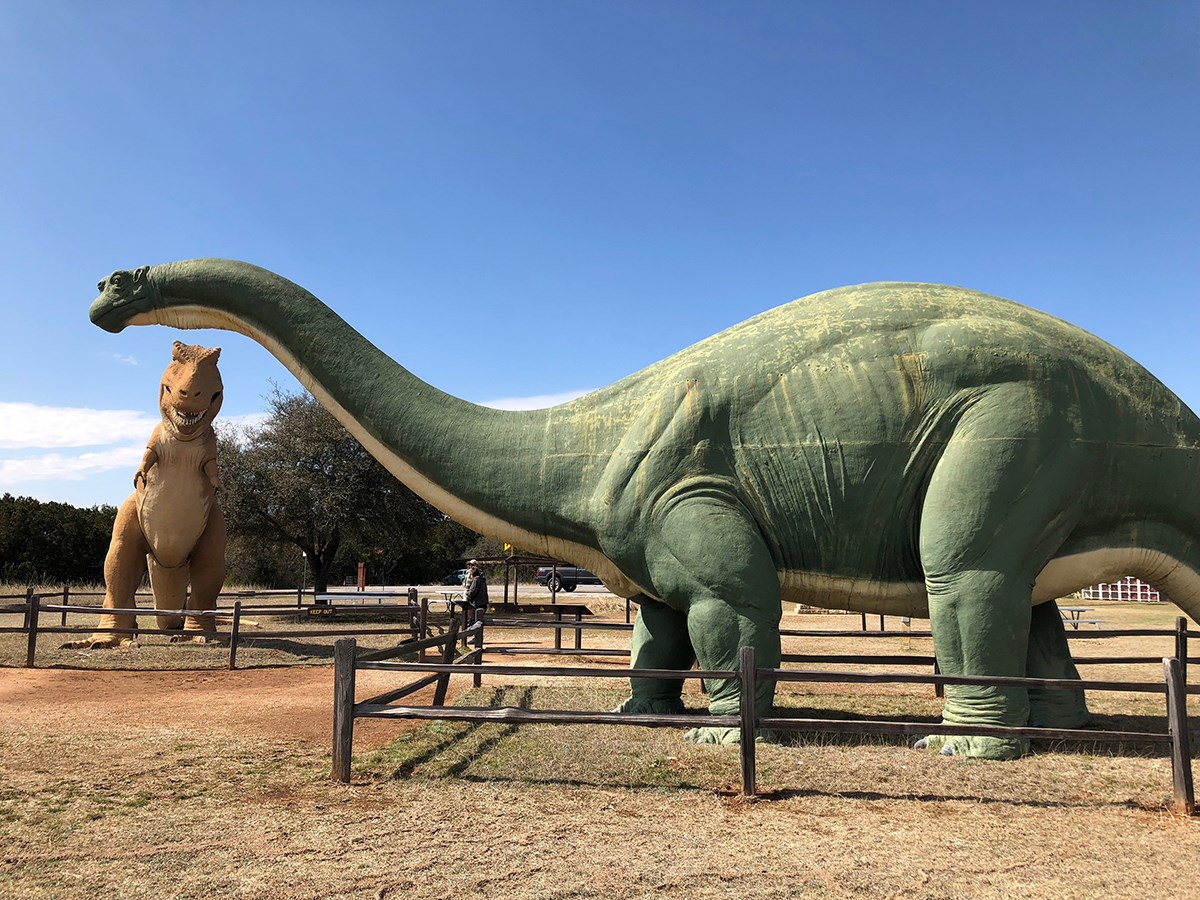This image depicts a scene from a dinosaur-themed park in the late fall to early spring in the United States, evident by the brown grass and bare trees in the background. The foreground features a large green Stegosaurus sculpture with a beige underbelly, enclosed by a rudimentary wooden fence. This dinosaur is easily identifiable by its long neck, large arched back, and thick legs. Adjacent to the Stegosaurus, another imposing dinosaur sculpture can be seen—a brown Tyrannosaurus Rex with a cream-colored underbelly. This T-Rex stands on two sturdy legs and faces the Stegosaurus, with its large teeth visible. Both sculptures are situated on an area of dirt or dried grass, with a rocky pathway leading up to them. In the distance, a parking lot with a vehicle can be spotted, emphasizing the outdoor setting and adding a touch of realism to this themed park scene.